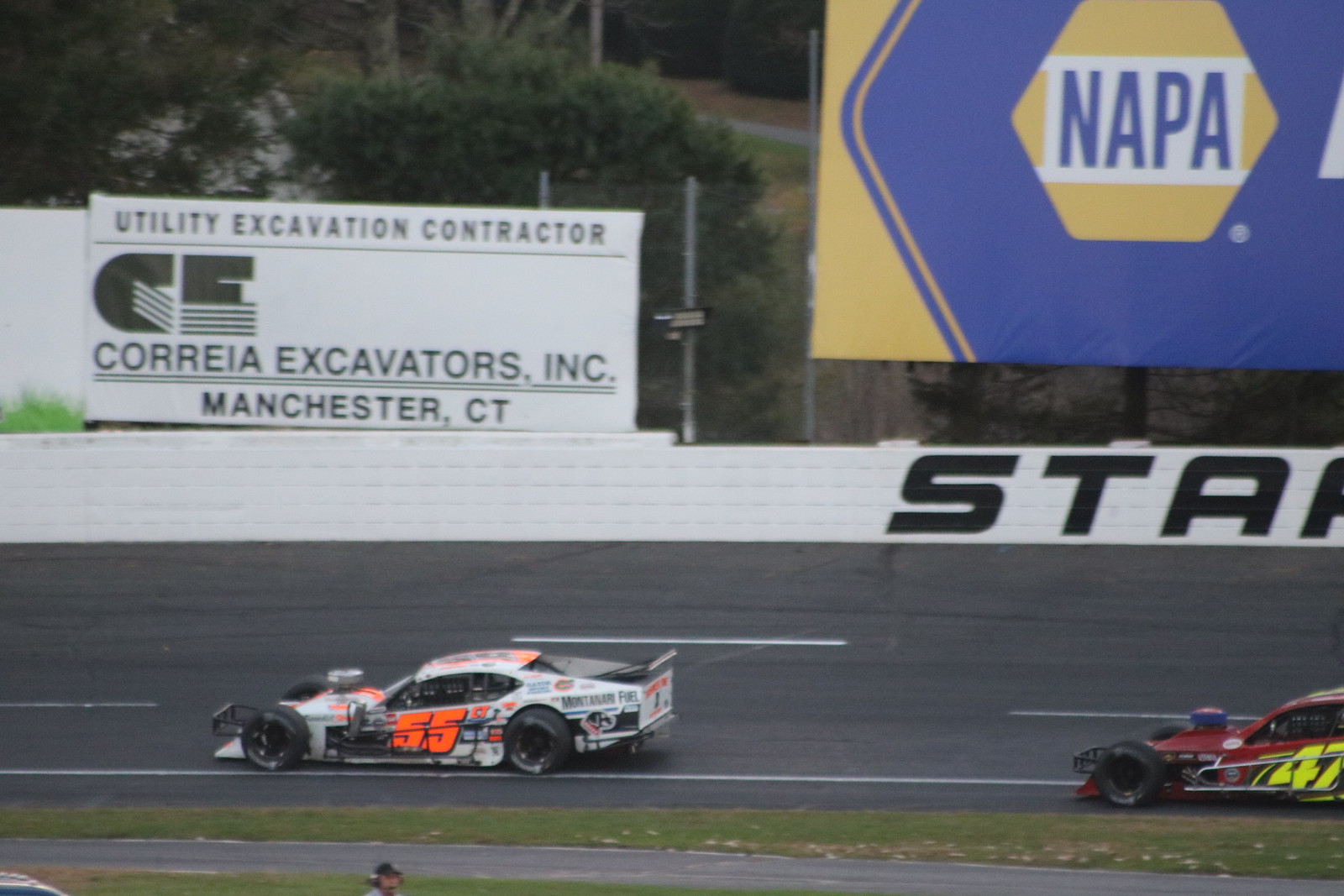The image captures an outdoor racetrack scene amidst a race. Dominating the foreground is a white car with black accents, adorned with fluorescent orange number 55 and multiple sponsorship decals. This vehicle is ahead of a dark red car, embellished with neon yellow number 47, which appears less sponsored. Both cars exhibit slight blurring, emphasizing their high-speed motion. The track is flanked by dense trees and a grassy area with a sidewalk. Prominent advertisements include a blue-and-yellow NAPA Auto Parts sign and a white board for Coria Excavators, Inc. from Manchester, Connecticut. The scene conveys the intensity and competition of the ongoing race.